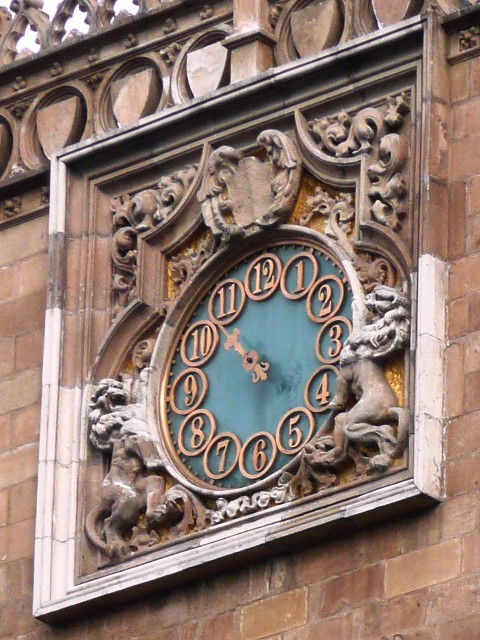This outdoor photograph features the facade of a stone brick building adorned with large, weathered bricks in varying shades of red, orange, and brown. Central to the image is a distinctive square frame housing an intricately designed clock. The clock face is green with gold circled numbers from 1 to 12 and gold hands, showing the time as approximately 10 minutes to 11.

Surrounding the clock are detailed carvings, including figures of animals walking on their hind legs on the bottom left and right, along with a shield-like shape with wings above it. Floral carvings and other ornate patterns embellish the area around the clock, adding to its historical and artistic appeal.

Above the clock, the building features additional decorative elements, such as small shield shapes set within circles and other pattern designs, culminating in an ornate stone ridge with looped arrowhead-like shapes at the top. The weathered appearance of the stone and the intricate details create a sense of timelessness and craftsmanship. An overcast sky peeks through at the top edge of the image, enhancing the ambiance of this architectural piece.